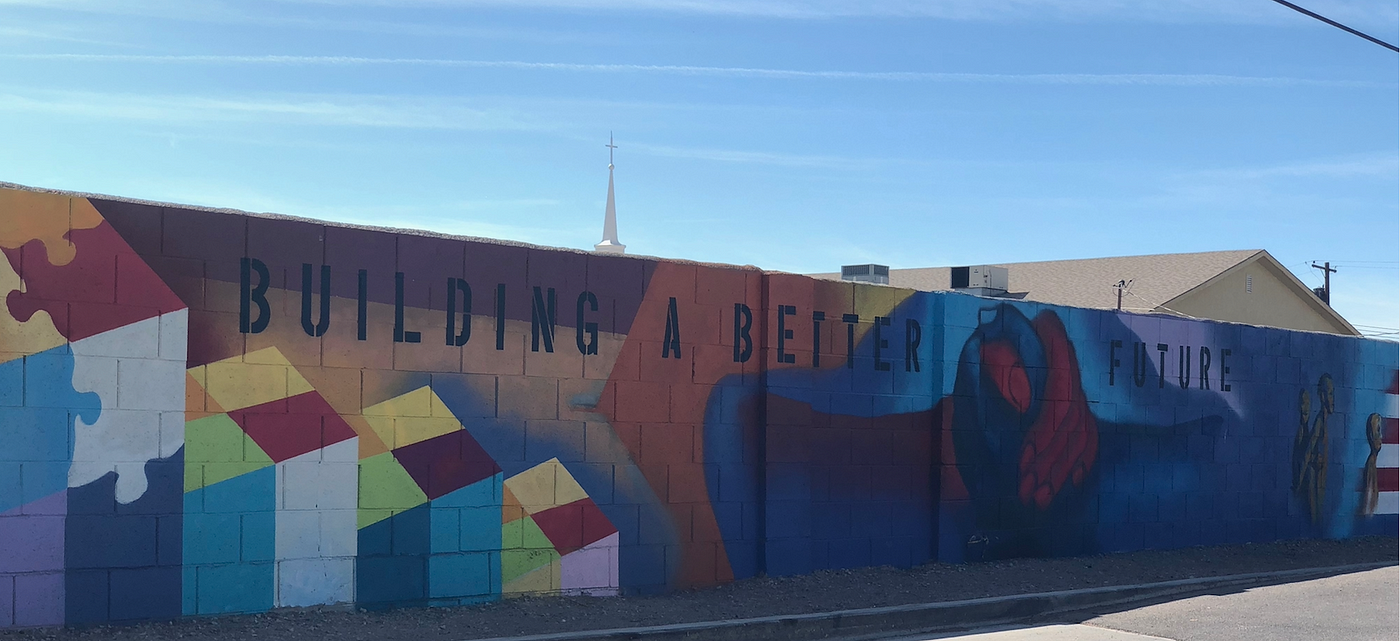The image features a large and expansive mural painted on a cinder block wall, extending almost half a city block and approximately two stories tall. Dominating the composition, black text runs across the top, declaring: "Building a Better Future." Below this inspirational message, the mural showcases colorful, puzzle-piece blocks arranged in a descending stair-like formation on the left side, reminiscent of Rubik's cubes. At the center of the mural, two clasped hands – one brown and one black – symbolize unity and cooperation, precisely positioned between the words "Better" and "Future." Surrounding the main imagery are vibrant swirls of blues, reds, browns, oranges, and yellows, adding a dynamic, abstract background to the scene. In the distance, behind the mural, a church building with a distinct steeple and cross is visible, placing the mural in a community setting.